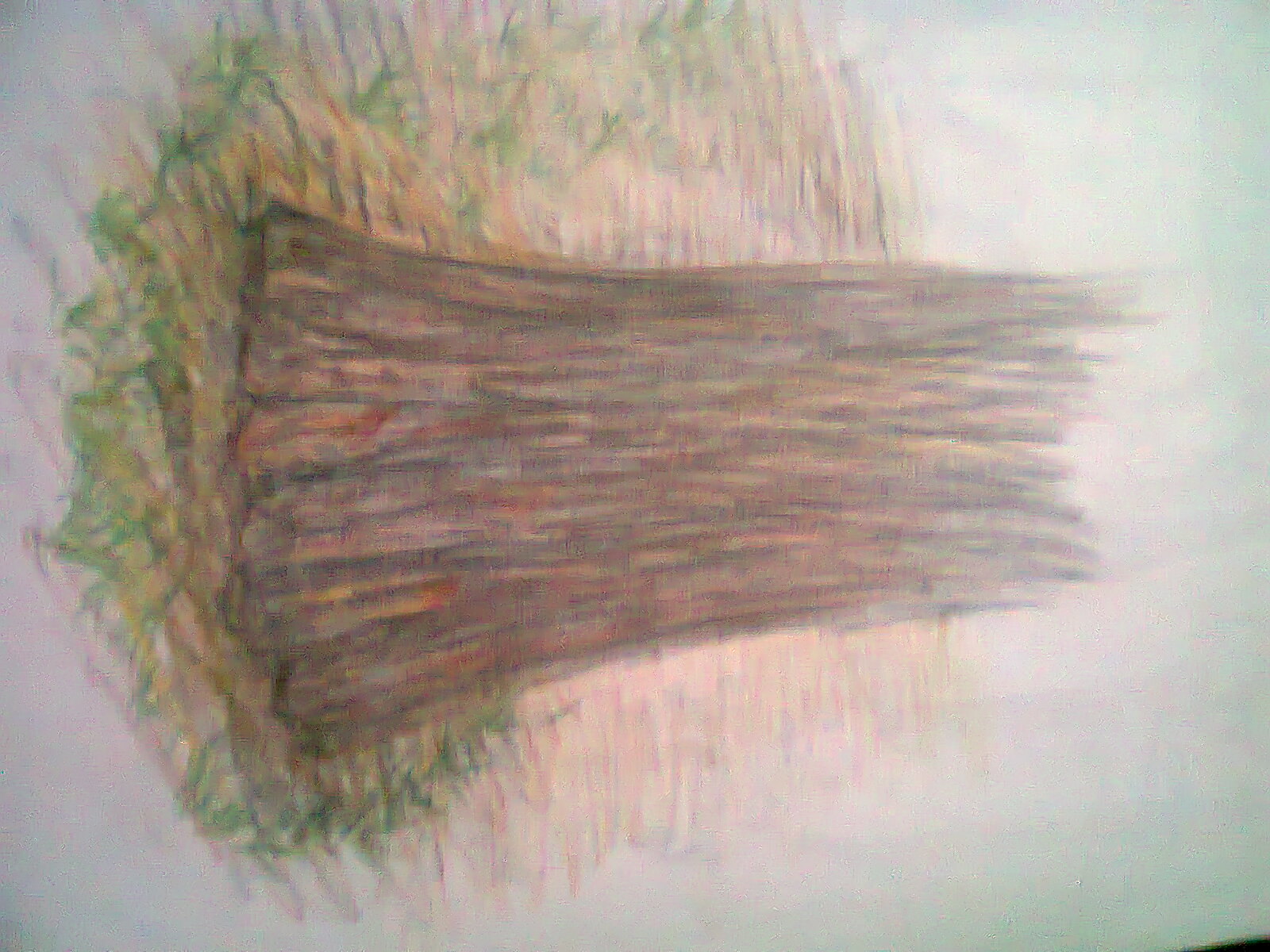This image showcases a child's colored pencil drawing, captured in a slightly blurry and sideways photograph. The focal point of the drawing, positioned centrally, is a tree trunk. This trunk, sketched in shades of brown, black, yellow, and perhaps a touch of rust, extends from the middle left towards the right. Surrounding the tree trunk on the left are hues of yellow and green, forming a somewhat chaotic circle, suggesting the ground or grass. The right side of the image, dominated by bright white and lightly colored background, appears to be overexposed due to a camera flash, creating an impression of a blue sky or possibly just an unintentionally bright area. Behind the trunk, soft colors of rust and pink can also be observed. The bottom right corner of the image features a small dark black sliver. Notably, the drawing lacks any branches, focusing solely on the tree's base and immediate surroundings, including indistinct lines and patches of orange, brown, and green at the trunk's base.